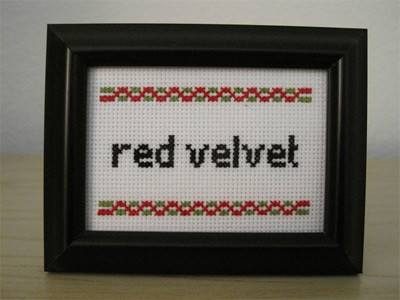The indoor image captures a black picture frame set on a light beige wooden table against a white wall. Inside the frame is a white canvas featuring intricate embroidery. The top and bottom edges of the canvas are adorned with a decorative border consisting of a red and green twisted rope pattern. Centered on the canvas, the phrase "Red Velvet" is prominently displayed in black lettering. The craftsmanship suggests a cross-stitch or crochet technique, possibly serving as an advertisement or a decorative piece related to 'Red Velvet.'